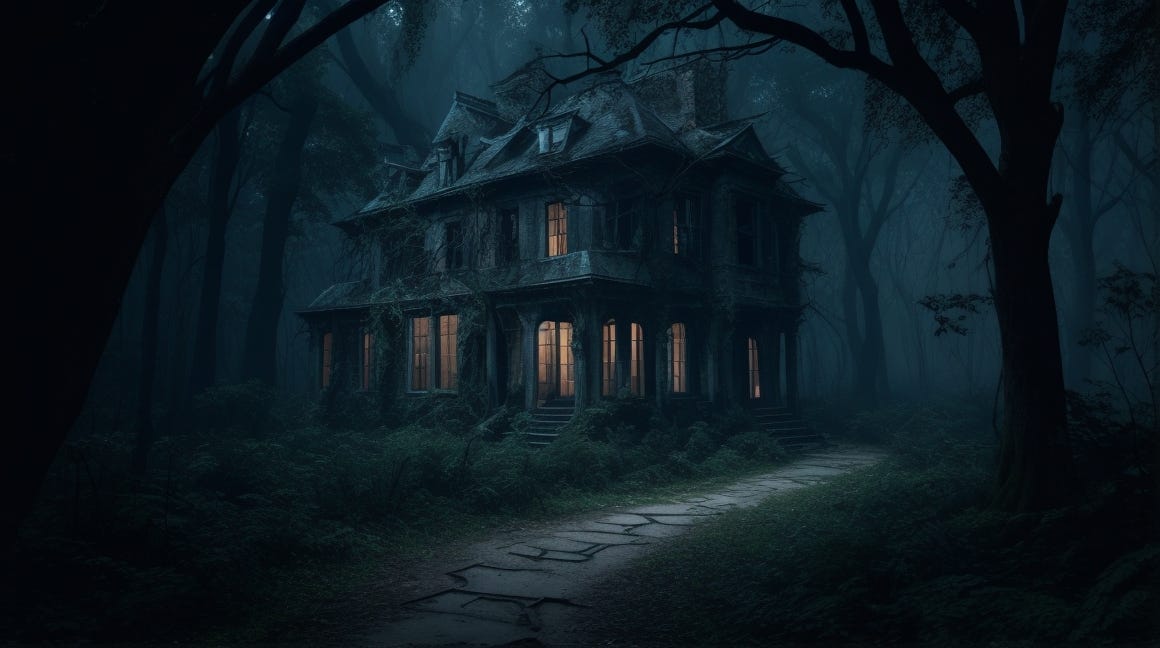The image portrays a spooky, old mansion situated deep within a dense, foggy forest, giving off an eerie, haunted vibe. At night, the scene is enveloped in darkness, punctuated by the faint glow of the moon high above, casting a light blue hue onto the treetops. The mansion itself is a two-story structure with an attic, all giving off a neglected appearance, with overgrown plants clinging to its walls. Several windows emit a warm, orange light, breaking through the gloom. A narrow, cobblestone path begins at the bottom center of the image, weaving through the dark woods toward the house. The left and right edges of the image are dominated by tall, black tree trunks, adding to the overall sinister atmosphere. In the foreground, particularly in the lower right corner, ferns grow amidst the grass, blending into the natural yet foreboding surroundings.